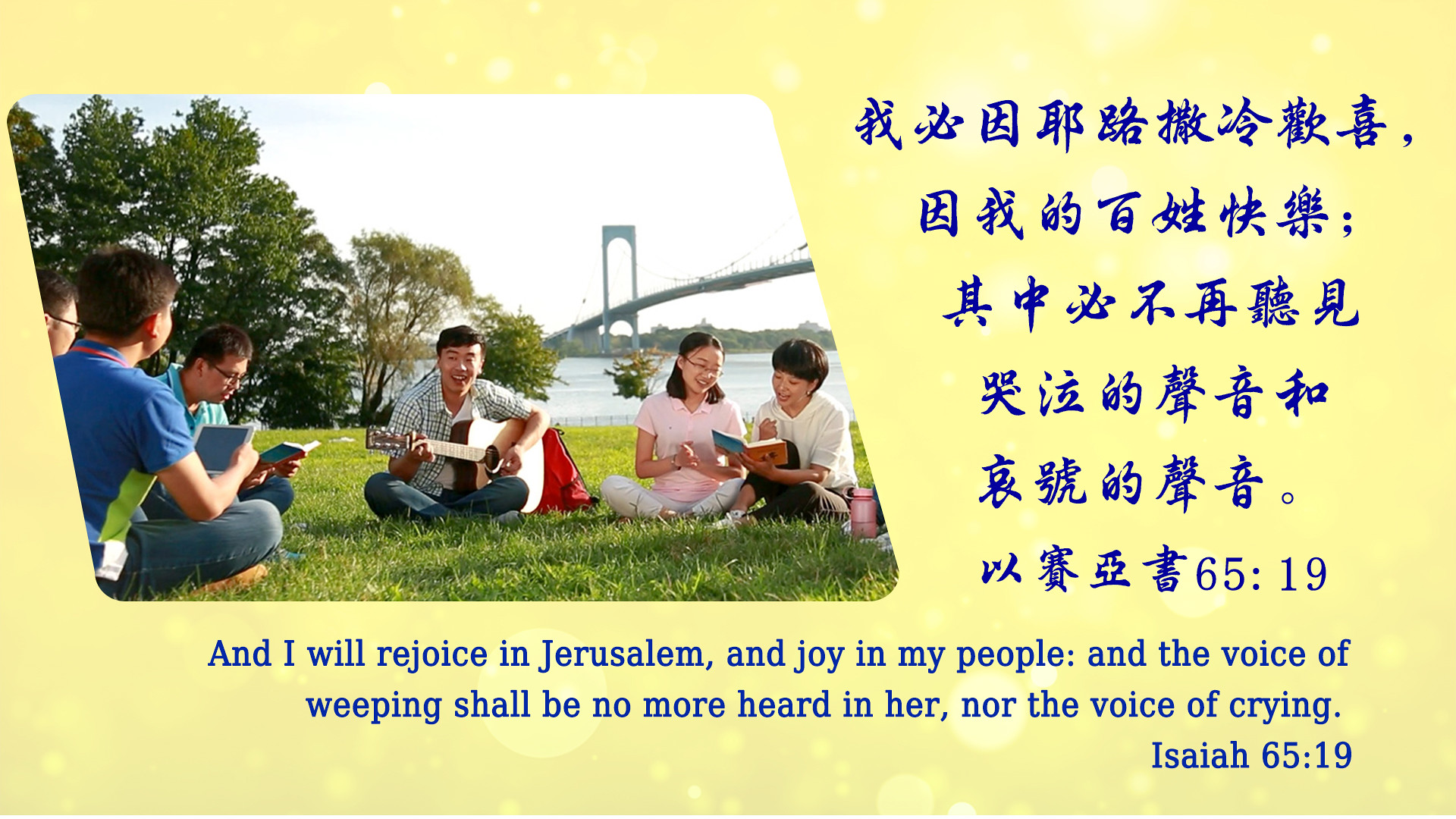The full-color printed card features a yellowish cardstock with blue print, adorned with a photograph. The text includes Asian characters which are accompanied by an English translation from Isaiah 65:19: "And I will rejoice in Jerusalem, and joy in my people. And the voice of weeping shall be no more heard in her, nor the voice of crying." The photograph captures an outdoor scene on a beautiful sunny day in a park, where a group of people of Asian descent are sitting on the grass. In the background, you can see trees, a body of water, and a long suspension bridge. One individual is holding a guitar, while the others are looking at books, likely songbooks. The imagery and text combined suggest a peaceful, joyful gathering.